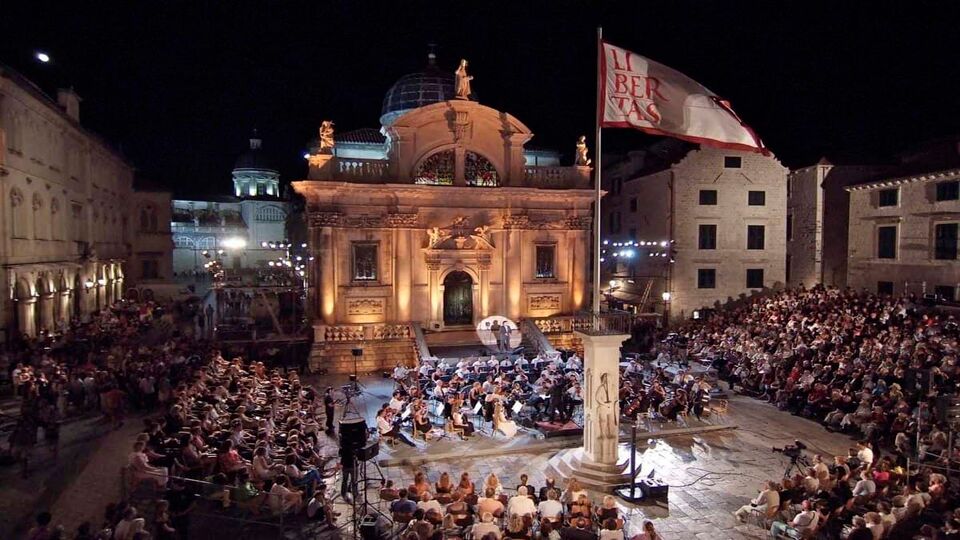The image captures a nighttime outdoor event, possibly an orchestral performance or public lecture, set in a city plaza surrounded by ancient-looking architecture. The focal point is a centrally illuminated building with distinct features reminiscent of Greek or Roman design, such as stone pillars and statues adorning the top. This building, which resembles a courthouse, has broad steps where a person stands under a spotlight, seemingly addressing the audience. In front of this building is an orchestra arranged in a U-shape with musicians sitting on chairs and possibly holding music sheets on stands. Surrounding the orchestra, there is a large, attentive crowd seated in rows of bleachers or standing. A prominent flagpole rises from a pedestal in the plaza’s center, displaying a white flag with red lettering spelling "Libertas." The entire courtyard is brightly lit, contrasting against the dark, black sky, highlighting the grandeur and historical ambiance of the setting.